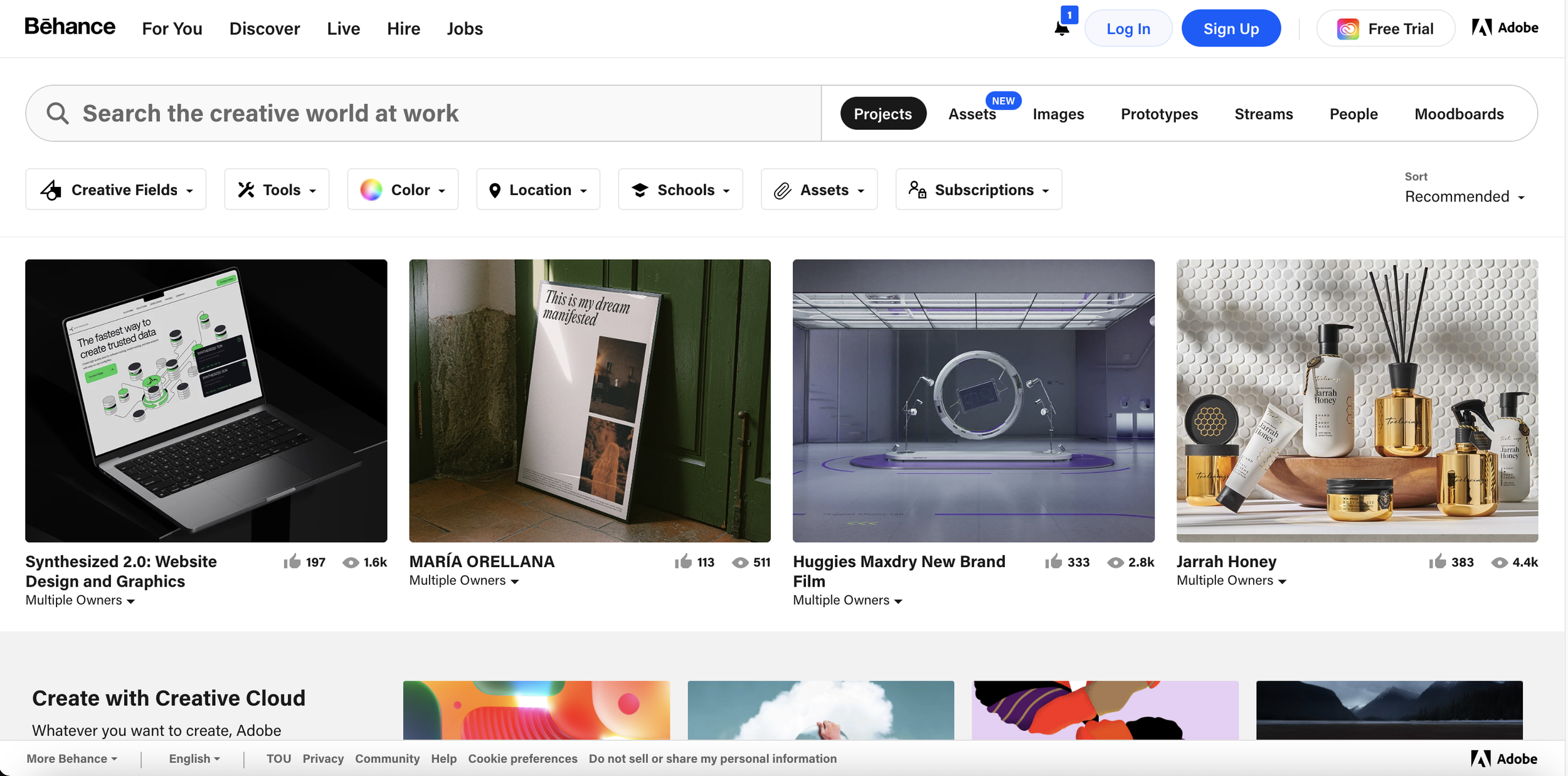This image showcases the homepage of the Behance website, a platform known for enabling users to discover, live stream, hire, and find jobs related to creative fields.

On the right side of the screen, there is an alert button accompanied by a blue box with the number "1" in the middle, indicating a notification. The main navigation area hosts options for logging in, which is highlighted with a light blue background, and signing up, which is highlighted with a dark blue background. There is also an option for a free trial, displayed on a white background along with an image of a square bearing pink, yellow, and blue colors, with "Adobe" written in the upper right-hand corner.

Below the navigation options, there is a prominently featured search bar encouraging users to "Search the creative world at work." The next section contains links to various categories such as 'Playlists,' 'Assets' (indicated by a blue circle with white text), 'Images,' 'Prototypes,' 'Streams,' 'People,' and 'Mood boards.'

Further down, the site highlights 'Creative Fields,' which includes various tools, a color wheel represented by a circle containing blue, yellow, and pink segments, 'Location,' 'Schools,' 'Assets,' and 'Subscriptions.'

The content section showcases an array of visual works:
1. The first image features "Synthesize 2.0," a project focused on website design and graphics.
2. The second image depicts "Maria Ordella," appearing to be a book propped up against a front door.
3. The third image highlights "Huggles, Madri," detailing a new brand film.
4. The fourth image is titled "Sarah Honey," displaying toiletries and mentioning multiple owners.

A board further down is labeled "Create with Creative Cloud," although the images associated with it are cut off in the view provided.